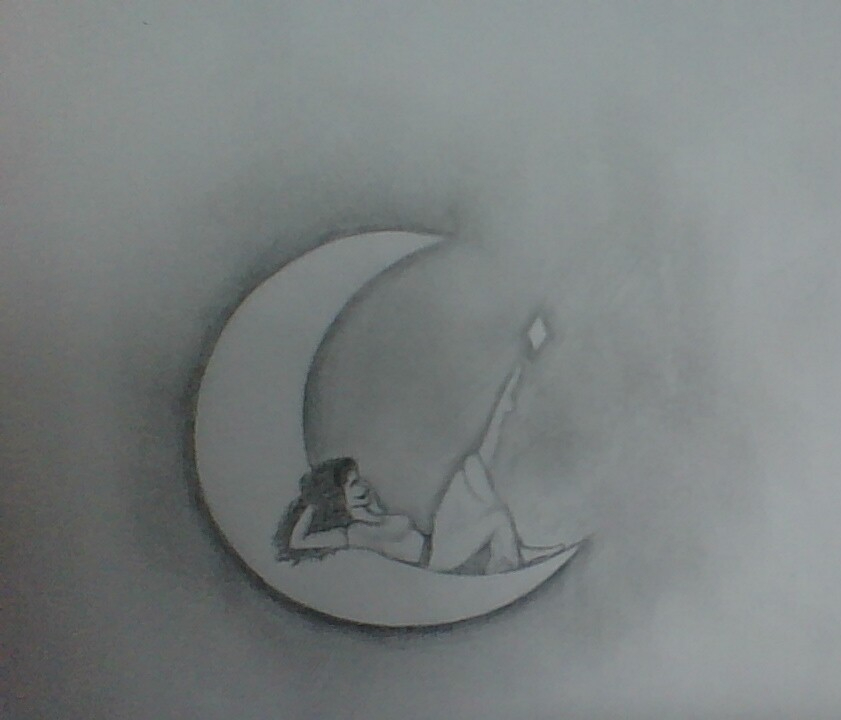This detailed, black-and-white pencil sketch depicts a young woman, seemingly in her 20s or 30s, reclining on the inner curve of a crescent moon. The background features a variety of gray shades, with some areas giving the impression of erased portions. The woman, with long, flowing black hair, is dressed in a short-sleeved dress with a belt and possibly a headband. She is smiling softly. Her arms are raised, touching her hair at the top. One of her legs, the left one, is elevated and pointing upwards, where her toes appear to touch a diamond-shaped star. The image, though somewhat crude and not deeply realistic, showcases a commendable level of skill and artistry.